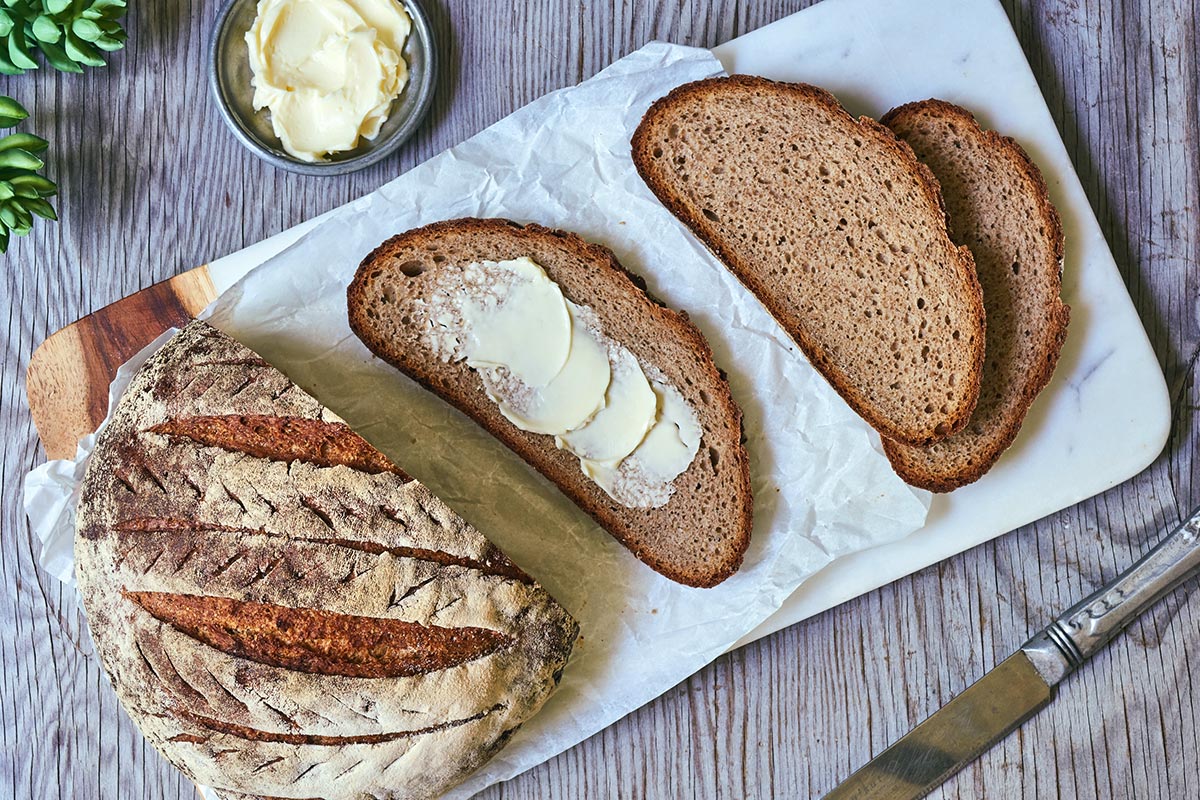The image shows a freshly baked, round loaf of wheat bread with a crispy crust, partially sliced and arranged on a white rectangular board with brown edges. This board is set diagonally on a brown wooden table, which is painted gray in areas. The loaf of bread, cut to reveal its soft, airy interior, sits in the center, with several slices neatly placed around it. 

Specifically, the left side of the board holds the larger, partially cut loaf, with the exposed, textured interior clearly visible. To the right of the loaf are three slices, one adorned with a smear of butter in the middle, but not reaching the edges. A silver bowl of butter is positioned in the upper left corner of the image, adding a metallic sheen. Completing the scene, a silver knife rests on the bottom right corner of the table, suggesting its use for cutting the bread and spreading the butter. The overall setting is visually appealing, inviting, and highlights the freshly prepared bread ready to be enjoyed.